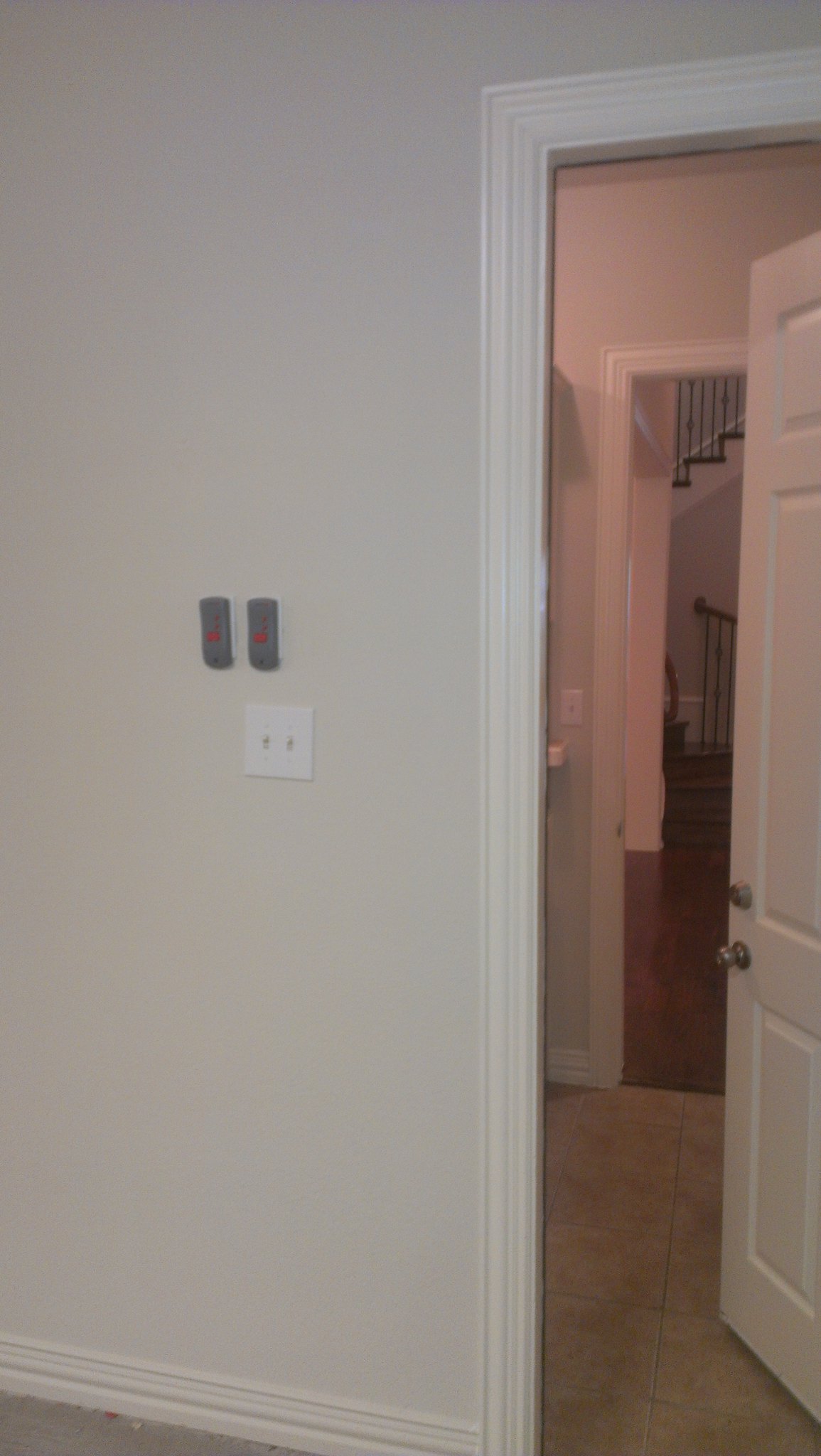This indoor photograph captures a serene snapshot of a home's interior, focusing primarily on a pristine white wall and a partially open door, leading the viewer's eye into adjacent rooms. The white wall is accented by a clean white wood trim along the floor and around the doorway. The door itself, also white, is fitted with a deadbolt lock and a doorknob, both featuring an elegant antique silver finish.

On this primary wall, there is a light switch, neatly framed by a white plate cover. The switches themselves are a matching white, with the left switch positioned upwards and the right one downwards. Mounted on the wall nearby are two mysterious grey plastic fixtures, each adorned with red buttons, hinting at an unspecified function.

Through the slightly ajar door, the image reveals a glimpse into the next room. At the far end, the viewer can discern another open door leading to a staircase that ascends upwards. Adjacent to this, there's an additional doorway—possibly part of a bathroom—where a small sink and another light switch are partially visible, adding a sense of depth and curiosity to the scene.